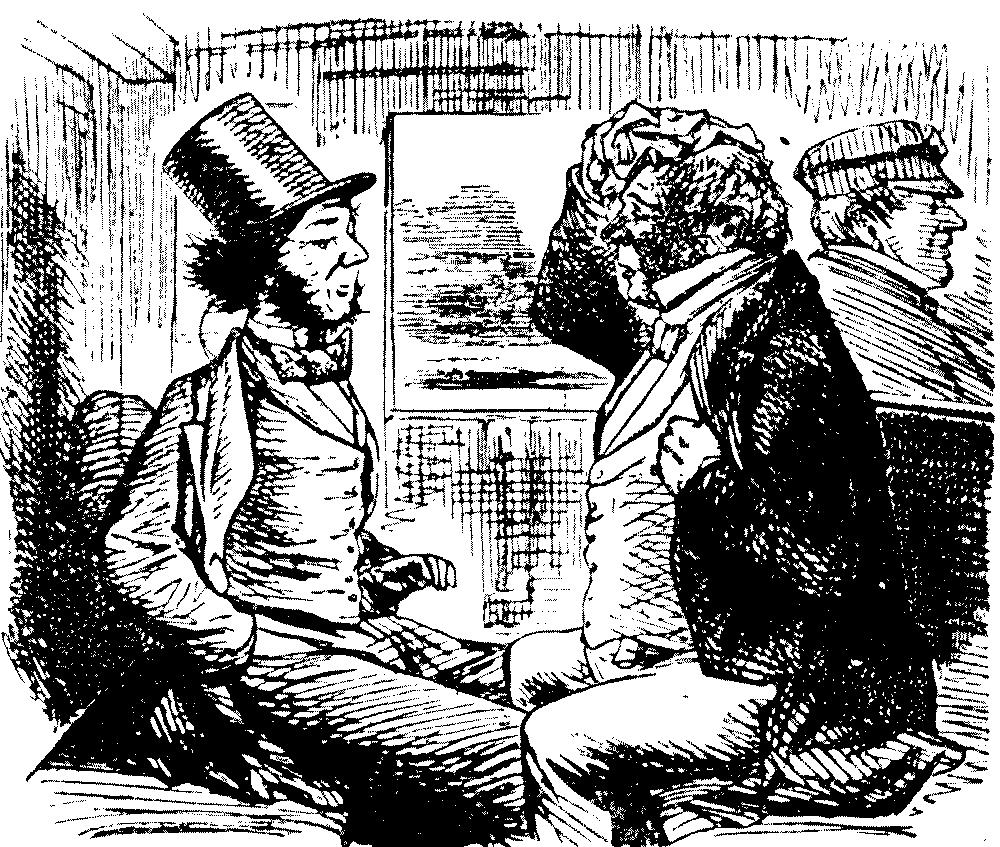This detailed black-and-white ink drawing, styled as an old-fashioned newspaper sketch with rough cross-hatching, depicts the interior of what appears to be a stagecoach or a train. Two men are seated on facing benches. The man on the left, thin with black hair and a beard but no mustache, is dressed in a top hat, a bowtie, a button-up vest, and a light-colored suit. He is engaged in conversation with the man opposite him. This seated man on the right is heavier, donned in a black jacket, vest, and pants, with a white collar and a bowtie. He is depicted holding a towel to his head, seemingly in pain. Behind him stands another man in profile, wearing an engineer's cap, reinforcing the setting as a train. A window behind them adds to the impression of motion, bringing the scene to life in this classic pen and ink illustration.